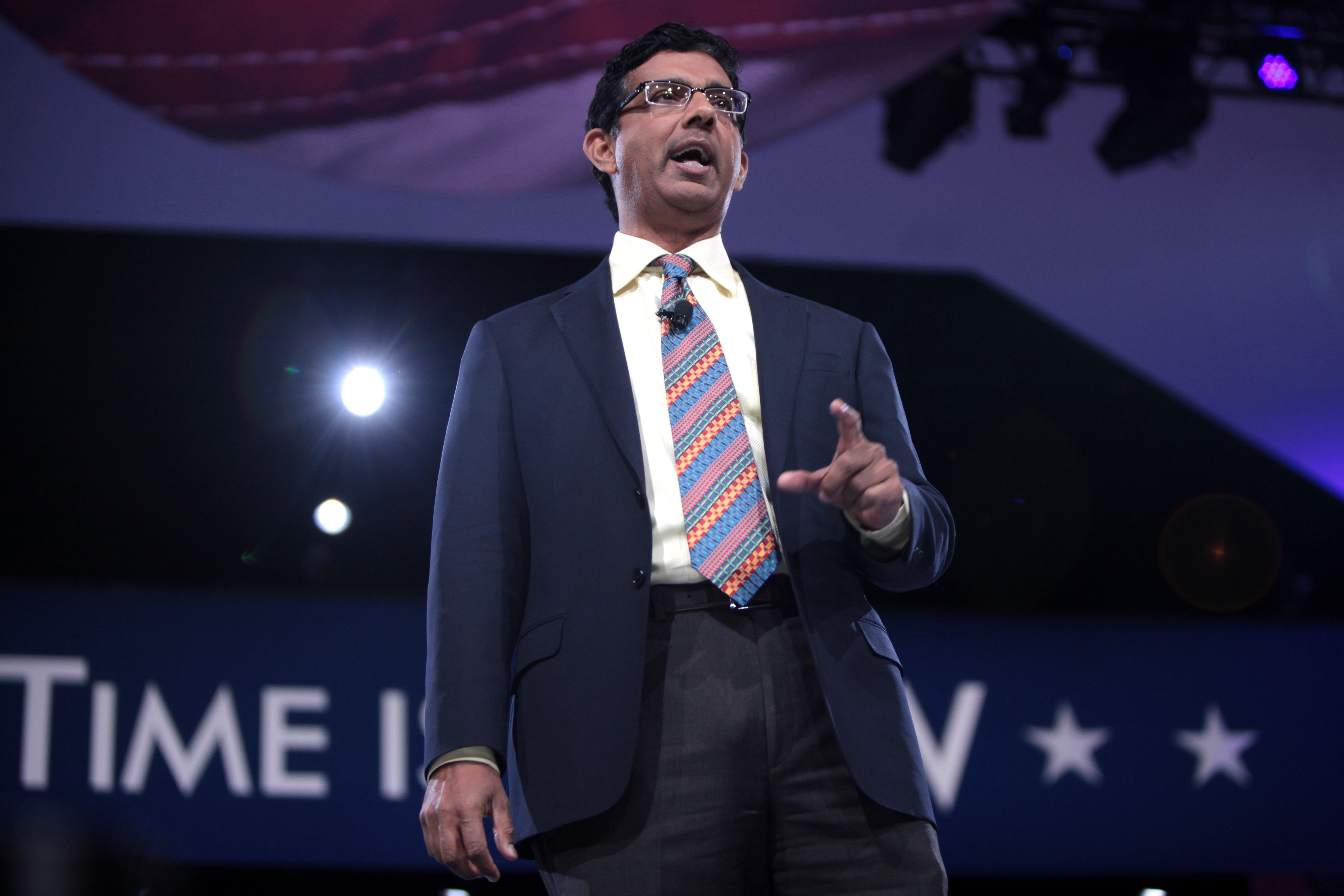This image captures a close-up, mid-length view of an Indian man who appears to be in his 40s or 50s, standing on a stage, possibly delivering a speech. He is positioned in the center of the frame, wearing a navy blue suit jacket over a white or cream-colored collared shirt, which is tucked into navy blue pants and secured with a black belt. His suit is complemented by a multicolored, striped tie featuring blue, red, and green hues, and there is a small microphone pinned to it. The man has short, wavy brown hair, square rectangular glasses, and is clean-shaven. He is gesturing with one hand, as if emphasizing a point. 

In the background, there is a predominantly black backdrop with various stage elements. On the left side of the image, a camera flash can be seen, and white stars are visible behind the man to his right. A white spotlight and additional stage lighting are present, contributing to the dramatic setting. The word "TIME" is partially visible in white letters at the bottom left corner, and there appears to be a navy banner and possibly a flag or ceiling decoration with white and red hues near the man’s head. This scene strongly suggests a formal or political event.